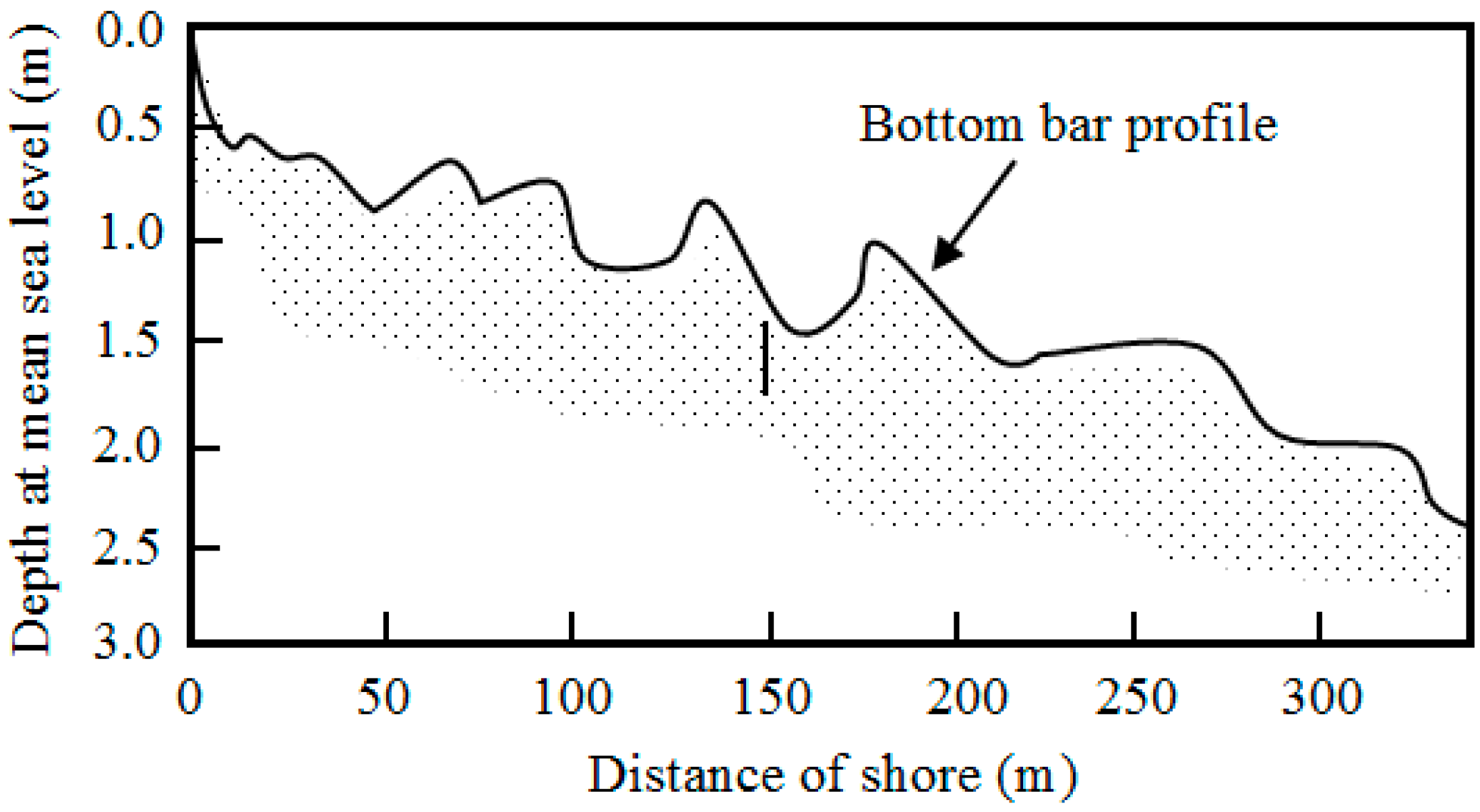The image is a black and white rectangular graph featuring a detailed depiction of depth at mean sea level against the distance from shore. The horizontal axis, labeled "Distance of Shore (M)," measures distance from 0 to 300 meters in 50-meter increments. The vertical axis, labeled "Depth at Mean Sea Level (M)," ranges from 0.0 at the top to 3.0 meters at the bottom, marked by increments of 0.5 meters. A prominent squiggly black line starts from the top left at 0.0 meters depth and descends toward approximately 2.5 meters on the right-hand side, resembling a mountain range. Positioned near the top right of the graph, the text "Bottom Bar Profile" is accompanied by a downward-pointing arrow directing attention to the line. Beneath this line are numerous smaller gray or black dots. All elements, including the axis labels and incremental markings, are rendered in black.